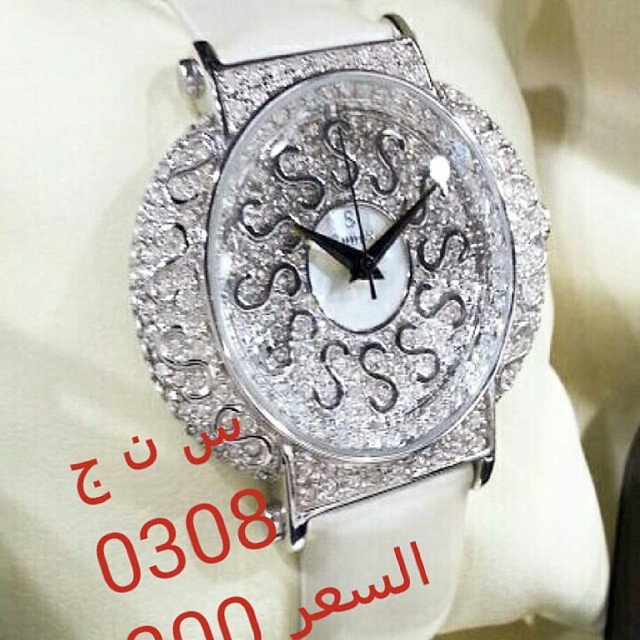The image depicts a glamorous wristwatch with an intricate design. The watch features a white leather band and is encrusted with sparkling diamonds all around its face. The face of the watch substitutes traditional numbers with the letter 'S' at every hour position, arranged in a clockwise circular formation. The watch has three hands: a long, thin black second hand, and shorter, thicker minute and hour hands. Surrounding the face are additional diamond embellishments, giving it an exceedingly luxurious appearance. The watch is set against a backdrop of a white pillow. There is red text with unrecognized symbols and the numbers "030A" and "0308," possibly in Arabic, adding a mysterious element.